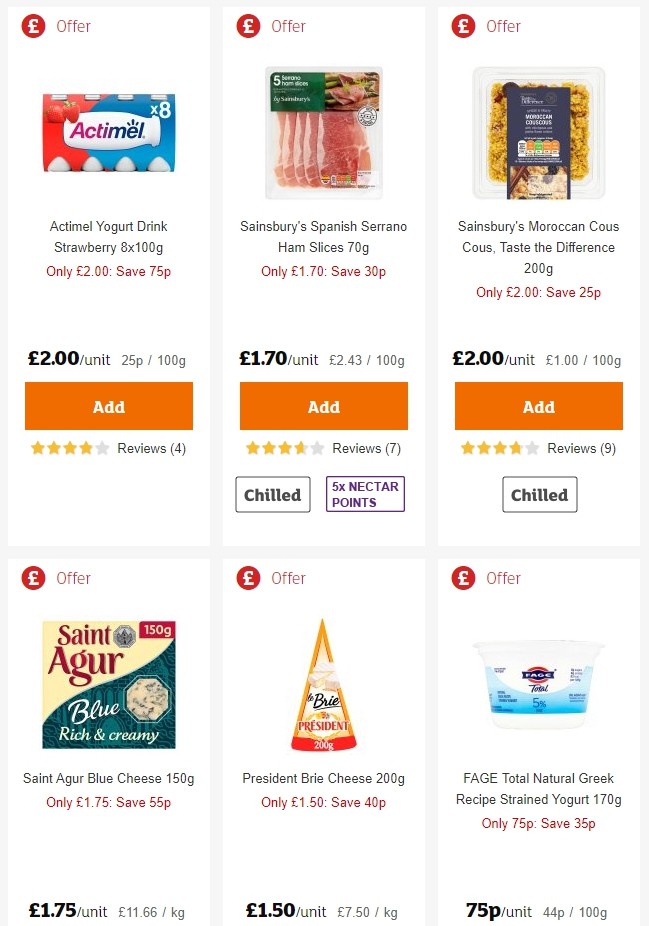The image depicts an e-commerce platform resembling an Instacart-style website displayed on a white background with grey borders separating the different sections. The interface showcases a variety of grocery items available for purchase, each accompanied by clear, high-resolution images. Featured products include Ossimel yogurt drink, various types of cheeses like blue cheese and brie, Moroccan couscous priced at two Euros, and slices of ham. The prices are listed in Euros, indicating that the website is tailored for a European market. Additional details such as product weight and refrigeration requirements are also visible, providing a comprehensive shopping experience.